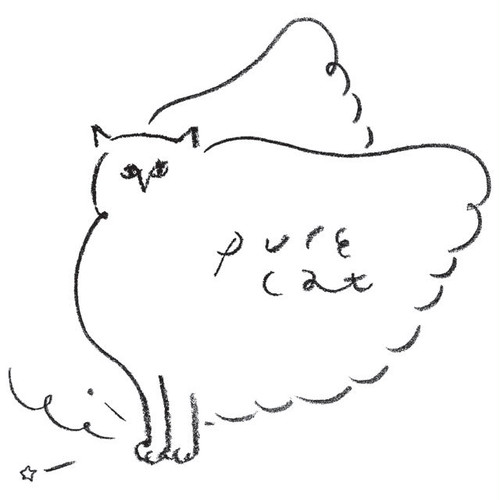The image is a simplistic, black pencil or charcoal sketch on a white background. Starting in the middle left-hand side, the outline of a cat is visible, featuring two pointy ears, and a face shaped in a circular oval with tiny eyes and a pointed nose. The drawing includes half of the cat’s body, rounded and ending with two paws at the bottom. Adjacent to the cat’s body, there is a large wing extending outwards, inscribed with the words "pure cat." Above the cat’s head, another partially occluded wing is discernible. Towards the bottom left of the image, decorative elements include the depiction of a shooting star and several curly lines. The cat, which has an owl-like face shape, is rendered in simplistic, crude line art, emphasizing its whimsical character.